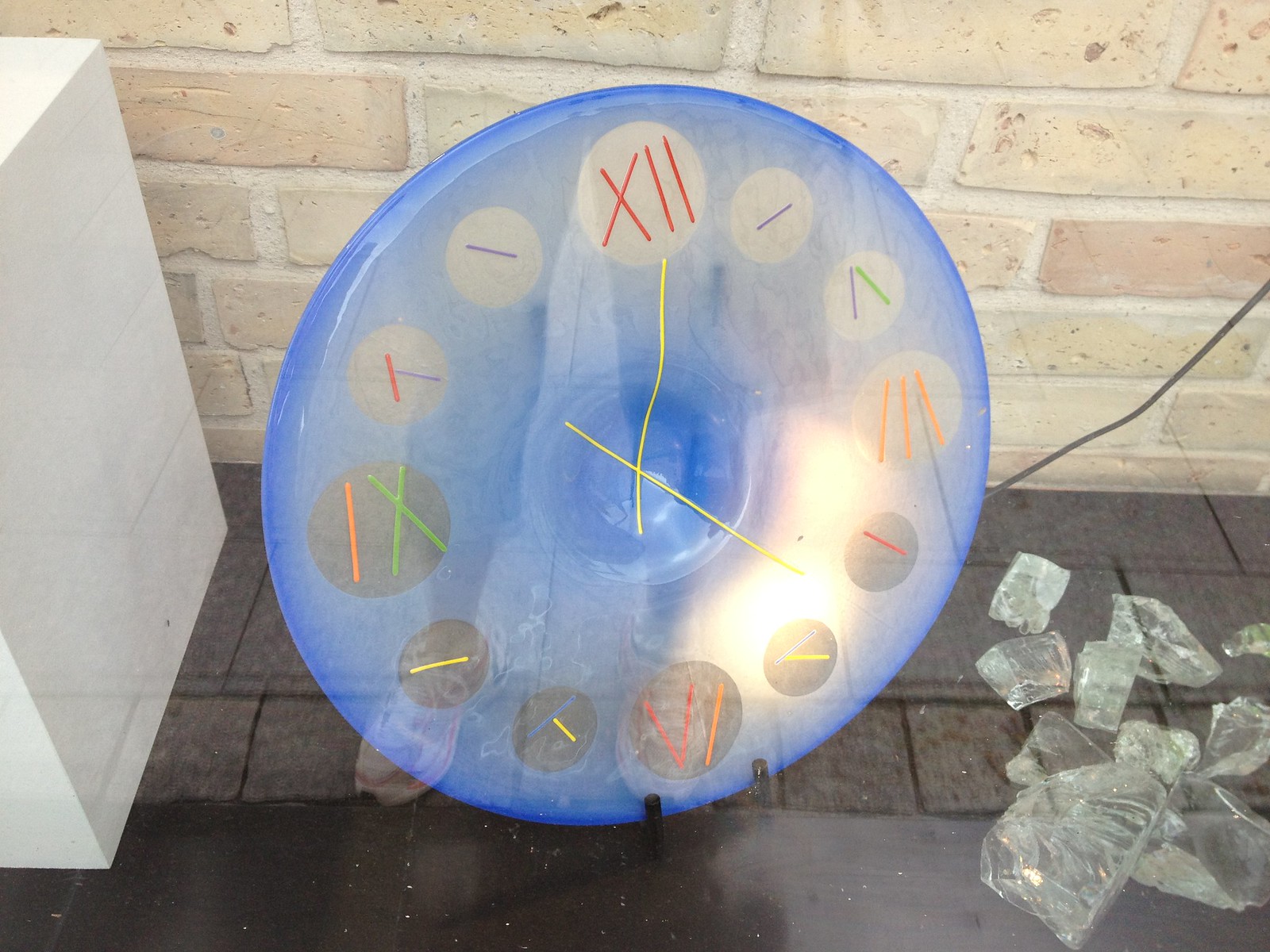A photograph captures a unique, Picasso-esque clock, featuring a whimsical mix of Roman numerals arranged in an unconventional pattern. Adjacent to the clock are translucent blocks resembling ice, though likely made of plastic, appearing shattered and fragmented. The clock, plugged in and illuminated, has a visible cord trailing from behind it. The scene is viewed through a pane of glass, with a subtle reflection of a woman’s feet clad in high-waisted pants visible in the lower portion of the image.